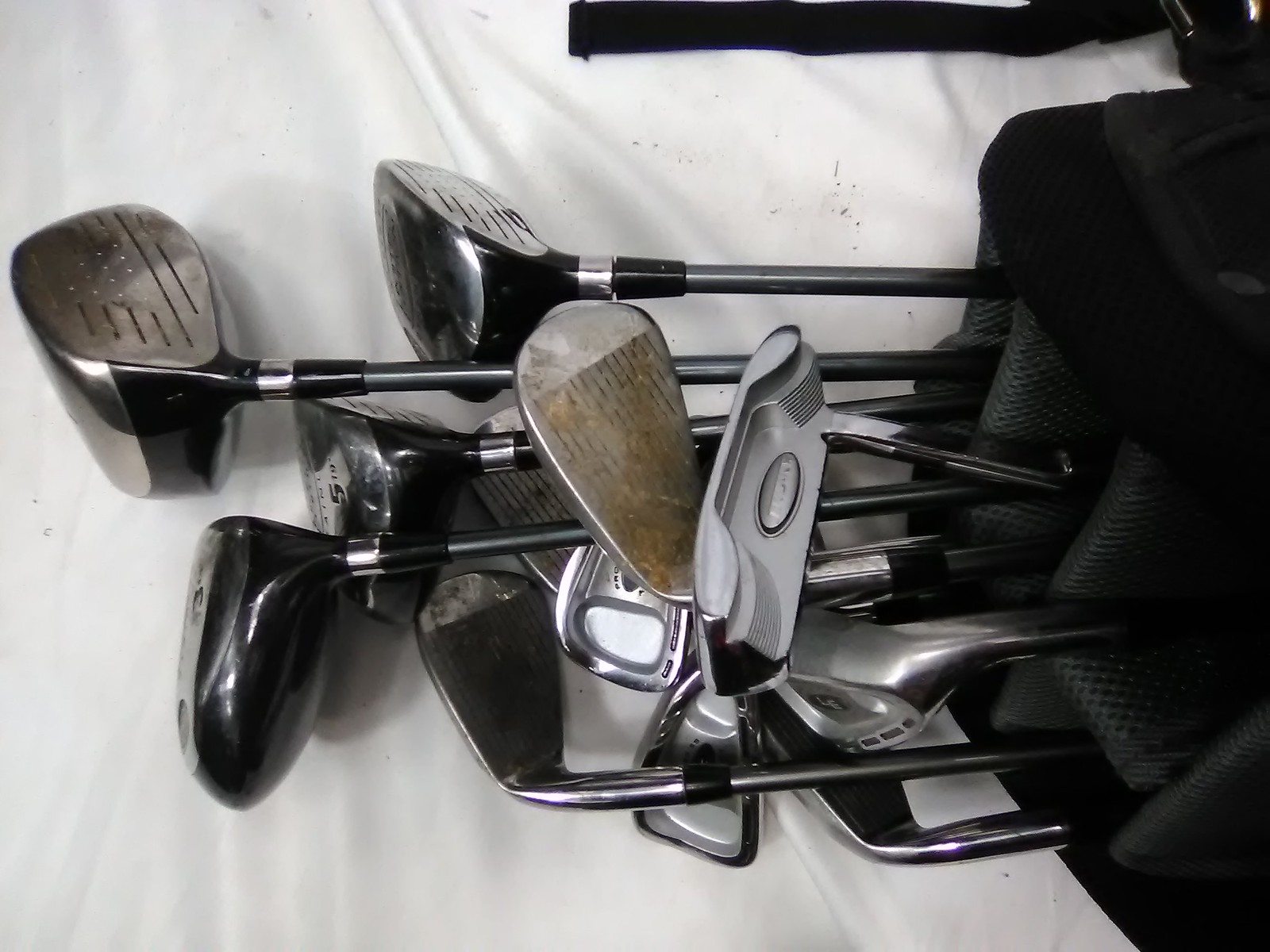The image depicts a well-used set of golf clubs, displaying clear signs of wear such as dirt and scuff marks on the club heads. These clubs are nestled in a black golf bag that appears to be made of black leather or fabric. The bag features divided compartments with a gray interior for organizing the clubs. Behind the clubs, a white cloth is visible, which has accumulated some dirt presumably transferred from the worn clubs. The bag's chrome handle and leather straps are also discernible in the image, and at least five to six golf clubs can be seen sticking out of the top, predominately in chrome and black finishes. The clubs share the spotlight with a couple of other gray matte finish metal objects that don't quite resemble typical golf clubs, adding an element of intrigue to the scene. The overall presentation is set against a white fabric background, which shows scattered debris, enhancing the impression of frequent use and outdoor activity.